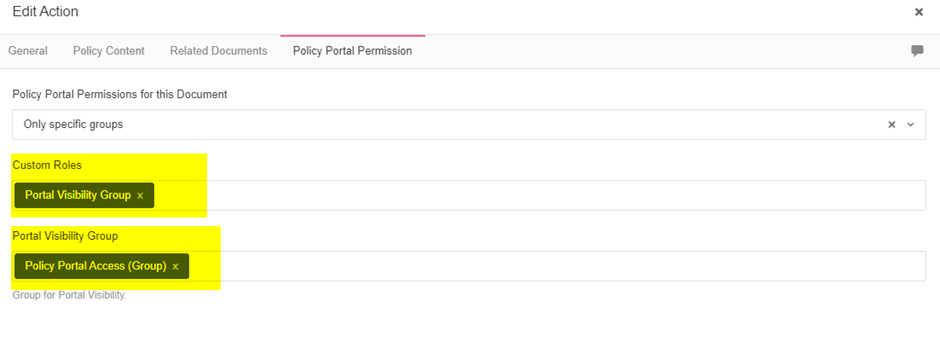**Caption:**

Screenshot of a webpage titled "Edit Action" showcasing multiple tabs at the top: General, Policy Content, Related Documents, and Policy Portal Permission (the active tab). A red line sits above the tabs. On the right side, there's a closeout cross and a comment box. Below, text boxes are present. The first box is labeled "Policy Portal Permissions for this Document" and contains another box within it stating "Only Specific Groups." There is also a closeout cross and a drop-down arrow to the right. Highlighted in yellow below this are sections for "Custom Roles" and "Portal Visibility Group," which can be collapsed using the black closeout cross. Another highlighted section in yellow follows with the label "Portal Visibility Group," where "Policy Portal Access (Group)" is mentioned in black. This section too can be closed with a cross. At the bottom is a combined group for portal visibility, tying back to the policy portal permission settings applicable to the document.